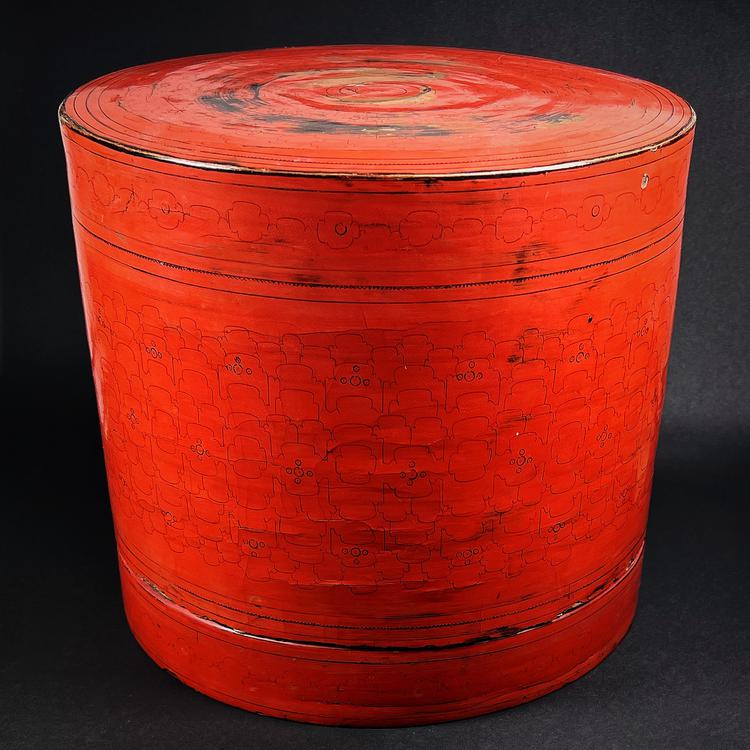The image is a photograph of a bright red cylindrical can, prominently positioned against a dark gray, carpeted surface. The exact dimensions of the can are ambiguous, leaving it unclear whether it is a handheld object or something larger like a barrel. The well-worn can displays dark scratches and areas where the red paint has chipped away, especially around the top, revealing some of the underlying metal in a visually pleasing, weathered manner. The can is adorned with intricate patterns resembling thin outlines of flowers and circular motifs, reminiscent of theater seat designs. The top of the can appears to have a cover, and the bottom edge shows slight damage with visible black smudges.